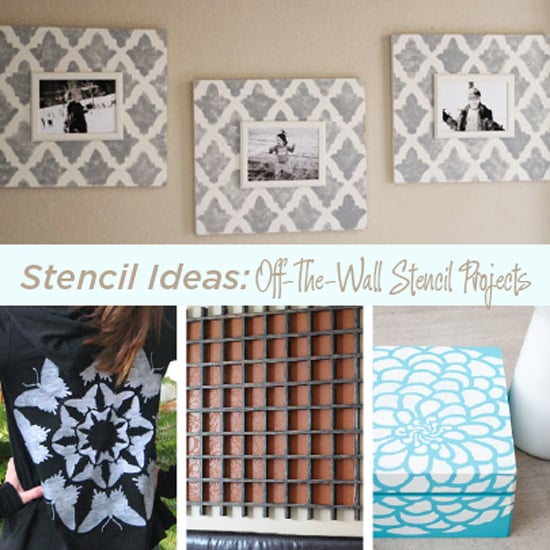This image showcases an advertisement for "Stencil Ideas: Off-the-Wall Stencil Projects." At its top, three black-and-white framed photos of people hang against a gray wall with a white crisscross and gray leaf-patterned background. Below these frames, the text "Stencil Ideas: Off the Wall Stencil Projects" appears in gray lettering, divided by a long white horizontal line. On the bottom left, there is a black shirt featuring a white star or snowflake design in the center, surrounded by silver butterflies. Centrally placed is a brown grid-style shelf or cover, demonstrating another stencil project idea. To the right, a blue and white floral-patterned gift box or container is displayed, and further right is a shirt adorned with white and black flowers, worn by someone. This image emphasizes the versatility of stencil projects, suggesting that stencils can be used for a variety of creative endeavors, from decorating shirts and storage boxes to making unique wall coverings and photo frames.